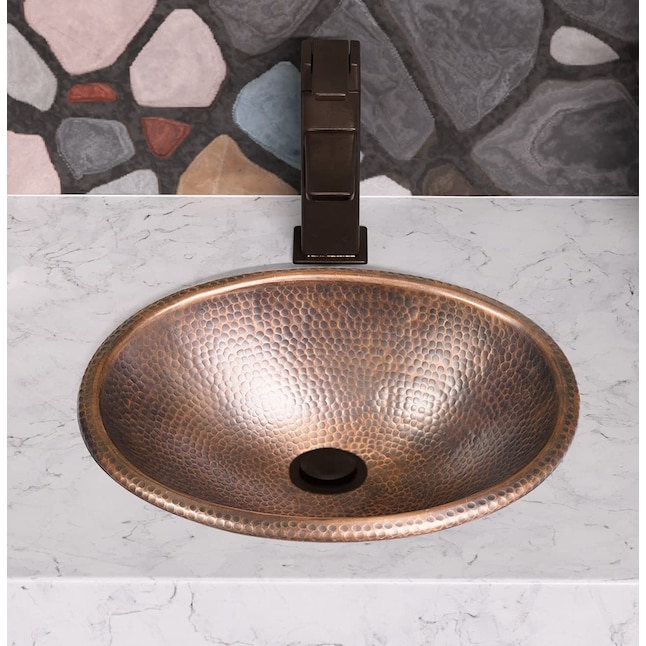This detailed, close-up image captures a modern bathroom vanity area showcasing a variety of elements. The countertop is constructed from pristine white marble with subtle gray veining, providing a sleek and elegant foundation. Prominently featured is a hammered copper sink with a unique, ornate design resembling scales or snake skin. This round, shallow basin gleams with a shiny, reflective surface, further accented by a black matte-finish drain plug at its center.

Complementing the sink is a sophisticated faucet positioned directly behind it. The faucet boasts a minimalist, modern design with a tall, straight spout and a single handle located at the top for straightforward operation. This faucet is also finished in a dark color, harmonizing with the sink's drain plug.

The backdrop to this setup is an eye-catching wall designed to mimic a stone mosaic. This backsplash includes an array of colors—dark gray, white, pink, light blue, and red—held together by wide black grout lines. Though the mosaic gives an impression of textured, protruding stones, it is actually an illustration or wallpaper, adding an artistic, contemporary flair without the bulk of real stones. This striking and cohesive design makes the vanity area an impressive blend of functionality and style.